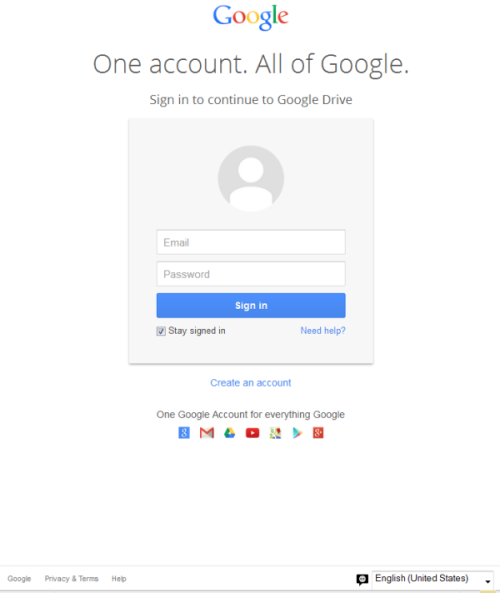The image appears to be a screenshot from a mobile device, displaying a Google sign-in page. The background is predominantly white. At the very top, bold and centered, is the word "Google". Below this, a tagline reads "One account. All of Google." prompting users to sign in to continue to Google Drive. 

Central to the screen is a rectangular, light gray section. At the top of this section is a user icon enclosed within a gray circle. Directly underneath, there are two white input fields; the first one labeled for email and the second for the password. Below these input fields is a prominent blue "Sign in" button. To the bottom left of this button, there is a checkbox accompanied by the text "Stay signed in." On the bottom right, in blue text, it states "Need help?".

Below the gray section, a blue "Create an account" link can be seen, followed by the statement "One Google account for everything." Further down, a row of icons depicting various Google services is visible: a blue square with a 'G' (Google account), a Gmail icon, a multicolored triangular "Google Drive" icon, a YouTube button, a Google Plus button, a possible Maps icon, and a Google Play button.

At the very bottom of the screen, a white border contains several text links. On the far left, it reads "Google," followed by "Privacy" and "Terms," then "Help". In the far right corner, "English (United States)" is displayed with a dropdown button beside it, suggesting language options.